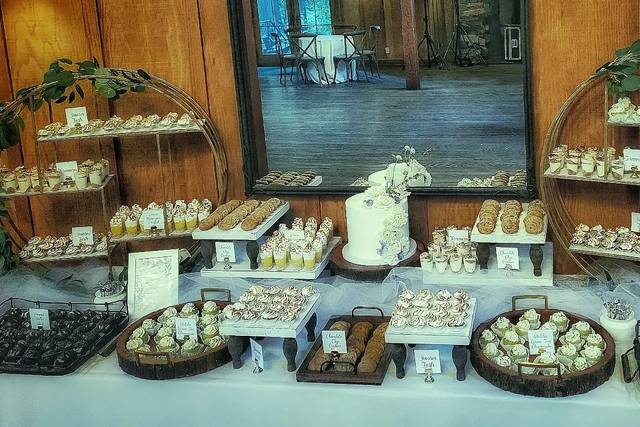The image showcases a lavish spread of desserts laid out on a table adorned with a white tablecloth. The backdrop is a wood-paneled wall featuring a centrally mounted mirror with a dark frame, which reflects the array of sweets including a prominent flat white cake adorned with flowers. The table is laden with an assortment of bakery delights such as mini cupcakes, cookies, possibly small donuts or eclairs, and other confectioneries. Each dessert is labeled with a white card held in metal holders, though the writing is too faint to read. At both ends of the table, there are stands with four shelves displaying additional treats. To the bottom-left of the image, a square tray holds chocolate cookies. On the top of the picture, there are circular trays decorated with leaves and an orange centerpiece surrounded by smaller desserts that could be mousse or gelato cups. The overall layout and decorations suggest a setting akin to a wedding reception. Additionally, the distant reflection reveals a hardwood floor and equipment such as a tripod-mounted speaker extending out of view.